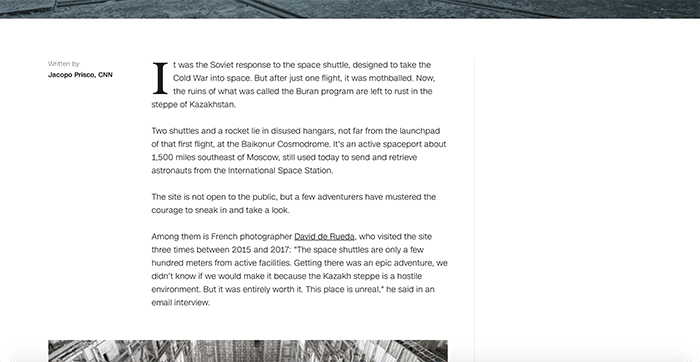In the image, the viewer sees a block of text, not in a communicative sense but as printed content, prominently featured. Across the top of the image, a gray banner stripe stretches horizontally. Below this banner, the image partially reveals what appears to be an apartment building, with a view looking down into a plaza or open courtyard area.

The text prominently states that Jacob Prisny of CNN wrote the article. The piece delves into the Soviet response to the American space shuttle program during the Cold War, specifically focusing on the Buran program. The Buran space shuttle, a USSR project designed to bolster the Soviet presence in space, completed only one flight before being abandoned. Now, the remnants of this ambitious program are left to decay in the steppes of Kazakhstan. The image evokes a sense of desolation and lost grandeur as it mentions two shuttles and a rocket lying forgotten in disused hangars near the Baikonur Cosmodrome's launch pad where that first and only flight took off.

The lower paragraphs of the text add further context, explaining that the site, though not open to the public, has drawn a few brave adventurers ready to risk sneaking in to witness the eerie remnants of this once-great Soviet space endeavor. The detailed narrative in the image portrays a poignant historical footnote, capturing both the ambition and the inevitable decline of this Cold War space project.